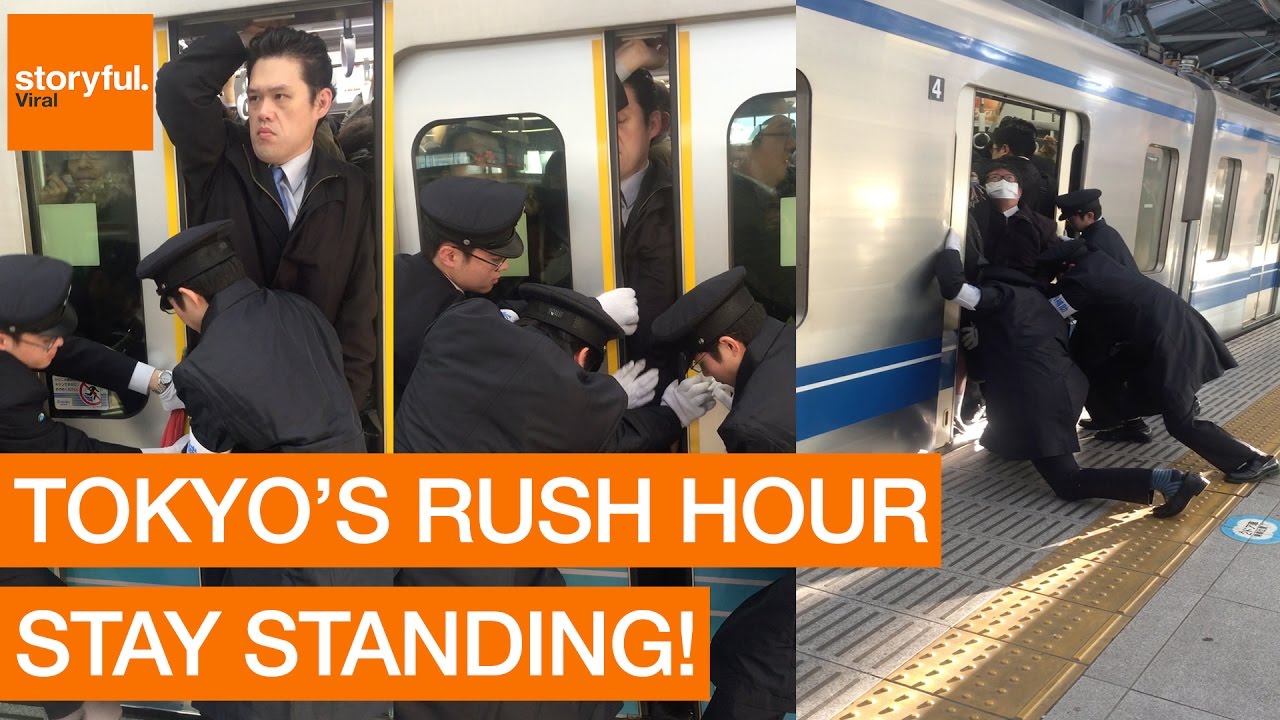This image, appearing to be a screenshot from the online news outlet "Storyful Viral," showcases a dramatic scene during Tokyo's rush hour. The top left corner features an orange square with the white text "Storyful" and the smaller black text "Viral" underneath. At the bottom, the caption "Tokyo's Rush Hour, Stay Standing" is displayed in white text within an orange bar.

The image is a composite of three consecutive photos. The first photo on the left shows a well-dressed man standing in the train doorway, reaching up to hold the door frame as two train operators attempt to push him inside and close the doors. The middle photo captures the moment as a third operator joins in, with the doors nearly shut. In the final photo on the right, the three operators are seen opening the doors, revealing a tightly packed crowd inside the train, with one noticeable masked man being pulled outward. The train appears to be slightly tilting to the right, emphasizing the intense crowding inside.